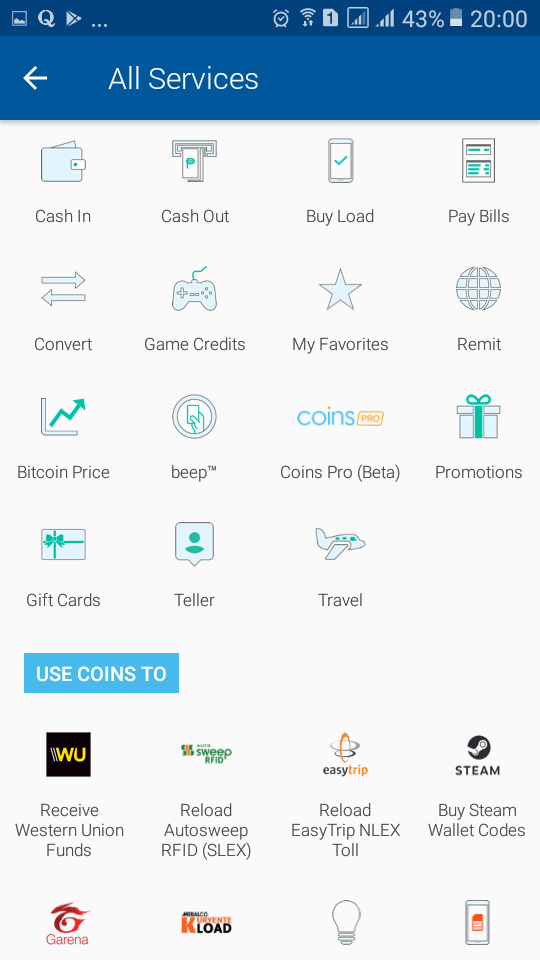The image depicts a cell phone screen displaying a list of service options in an organized, detailed interface. At the top of the screen, there is a dark blue header with essential icons: on the left are three cell phone icons, while the right shows multiple symbols including Wi-Fi, an alarm clock, a connection indicator, the battery percentage at 43%, and the time displayed as 20:00.

Just below the dark blue header, on a lighter blue background, the section labeled "All Services" is prominently displayed in white text with an arrow pointing to the left. The main interface, comprising the majority of the screen, is organized into categorized service options presented in rows and columns.

The first row features options such as "Cash In," "Cash Out," "Buy Load," and "Pay Bills." The second row continues with "Convert," "Game Credits," "My Favorites," and "Remit." Moving further down, the third row includes "Bitcoin Price," "Beep," "Coins Pro," and "Promotions." The subsequent row lists "Gift Cards," "Teller," and "Travel."

Below the primary list of services, enclosed in a light blue rectangle, there is an additional instruction that says "Use Coins To," followed by specific functions like "Receive Western Union Funds," "Reload," "Auto Sweep RFID," and "Reload Easy Trip Anilyx." Adjacent to these, another option indicates the ability to "Buy Steam Wallet Codes," supplemented by four additional icons below this segment.

The image concludes with a predominantly white background occupying the lower 85% of the screen, providing a clean and easy-to-navigate visual layout for users browsing through the numerous service options available on their cell phone.